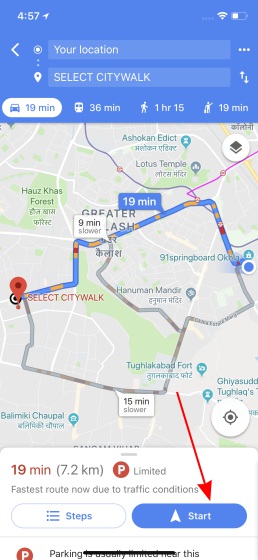The image is a screenshot from a cell phone displaying a map application. At the top of the screen is a blue status bar featuring the time, "4:57," in white, alongside icons for WiFi and battery status. Below the status bar, also within a blue band, there are text boxes with white text. The first text box indicates "Your Location," and the second one designates the destination as "City Walk."

An arrow icon for navigating back out of the app is also present within the blue band. The screen details various travel times to City Walk, showing 19 minutes by car (highlighted in blue ink over a white text box), 36 minutes by bus, 1 hour and 15 minutes if walking, and 19 minutes if hitchhiking. All other times are displayed in white ink against the blue band background.

Below these time estimates is a map illustrating the route to City Walk, including a red arrow pointing towards text that says "Stats," written in white over a blue text box.